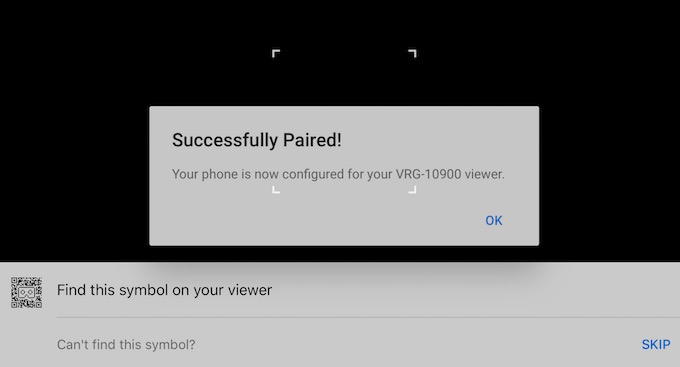The image displays a predominantly black screen featuring a user interface for pairing a device. At the center, there's a QR code used for scanning, reminiscent of those seen in camera roll functionalities. Surrounding the QR code are four dots, framing a gray pop-up box. This box contains black text reading, "Successfully paired!!!" below which, in gray text, the message, "Your phone is now configured for your VRG-10900 viewer." is visible. 

At the bottom right-hand corner of the screen, a blue "OK" button is positioned. Below this, there is a thin black strip followed by another gray box stretching across the width of the screen. Within this second gray box, there is another QR code with the instruction, "Find this symbol on your viewer." A faint gray line extends horizontally to the edge of the screen. Beneath this line, gray text reads, "Can't find this symbol?" In the bottom-right corner, blue text in capital letters states, "SKIP."

Overall, the interface clearly guides the user through the pairing process with visual cues and user-friendly text placements, ensuring a straightforward and efficient setup for the VRG-10900 viewer.